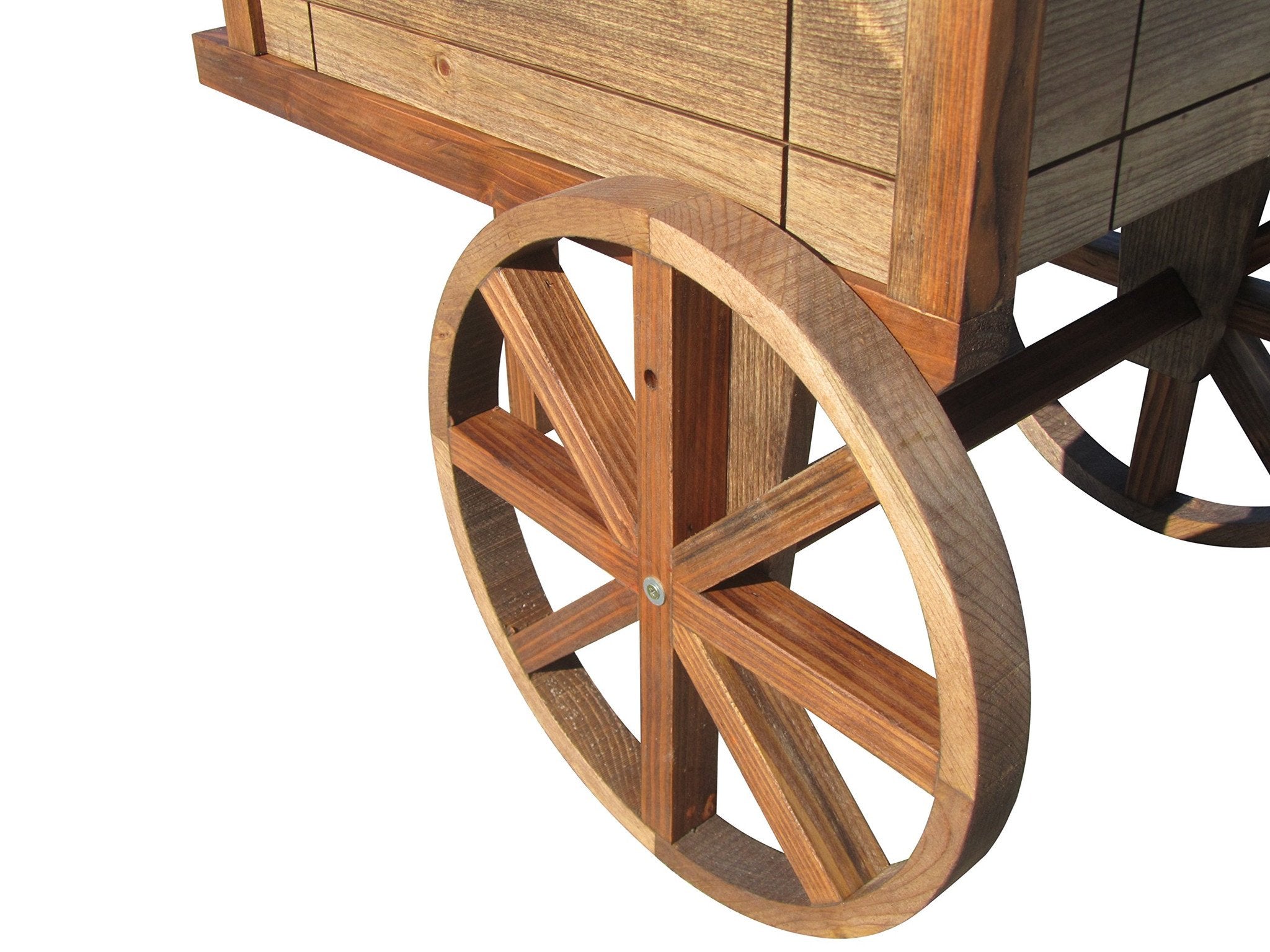The image is a detailed, close-up illustration of a wooden cart or wheelbarrow set against a completely white background. The focal point is on the wheel and part of the cart, with a full wooden wheel prominently in the center. The wheel itself is constructed from four curved sections of bent wood, joined together with square-stock wooden spokes. The cart wheel shows a contemporary metal screw and washer securing its components.

In the top right corner of the image, a corner of the wooden cart pops out into view. Along the top half of the photo, parts of the cart are also visible. The light wood of the cart suggests recent construction. Additionally, the axle connecting to another partially visible wheel is observable, with about one-third of this secondary wheel and its shadow also present. The overall scene is static, with the cart appearing completely still. The composition of the cart highlights its entirely wooden structure except for the modern metal fasteners, capturing the traditional yet contemporary craftsmanship.